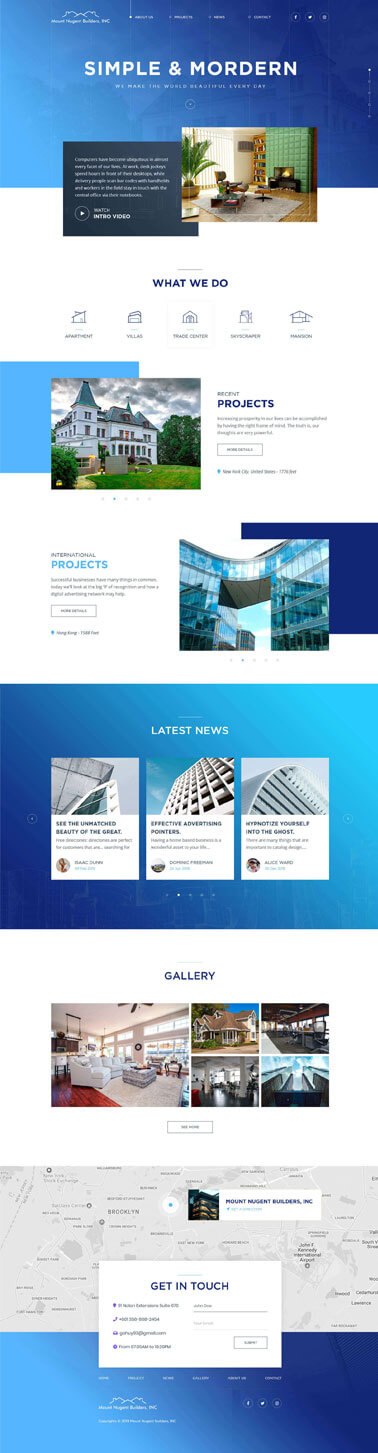The image depicts a webpage layout for a website titled "Simple and Modern," prominently displayed at the top center. The screen is composed of a series of blue and white panels arranged in an alternating pattern from top to bottom, with various images superimposed to draw attention to different sections.

Starting at the top, there is a blue panel followed by a grey one displaying a picture. Below this, a white panel prominently features the text "What We Do" at its center, accompanied by several icons that can be clicked for more detailed information. Next, another blue and white panel is present with a superimposed image of a house, highlighting the projects they undertake.

Following this is a similar blue panel with another inset image, showcasing additional projects. The center of the layout includes a full-width blue panel displaying three images of modern skyscrapers alongside a section titled "Latest News."

Further down, yet another blue panel features three more images of buildings and skyscraper views. At the bottom of the webpage, there is a section resembling a map, followed by a blue section and a central white panel providing contact information and various methods to get in touch with the website operators.